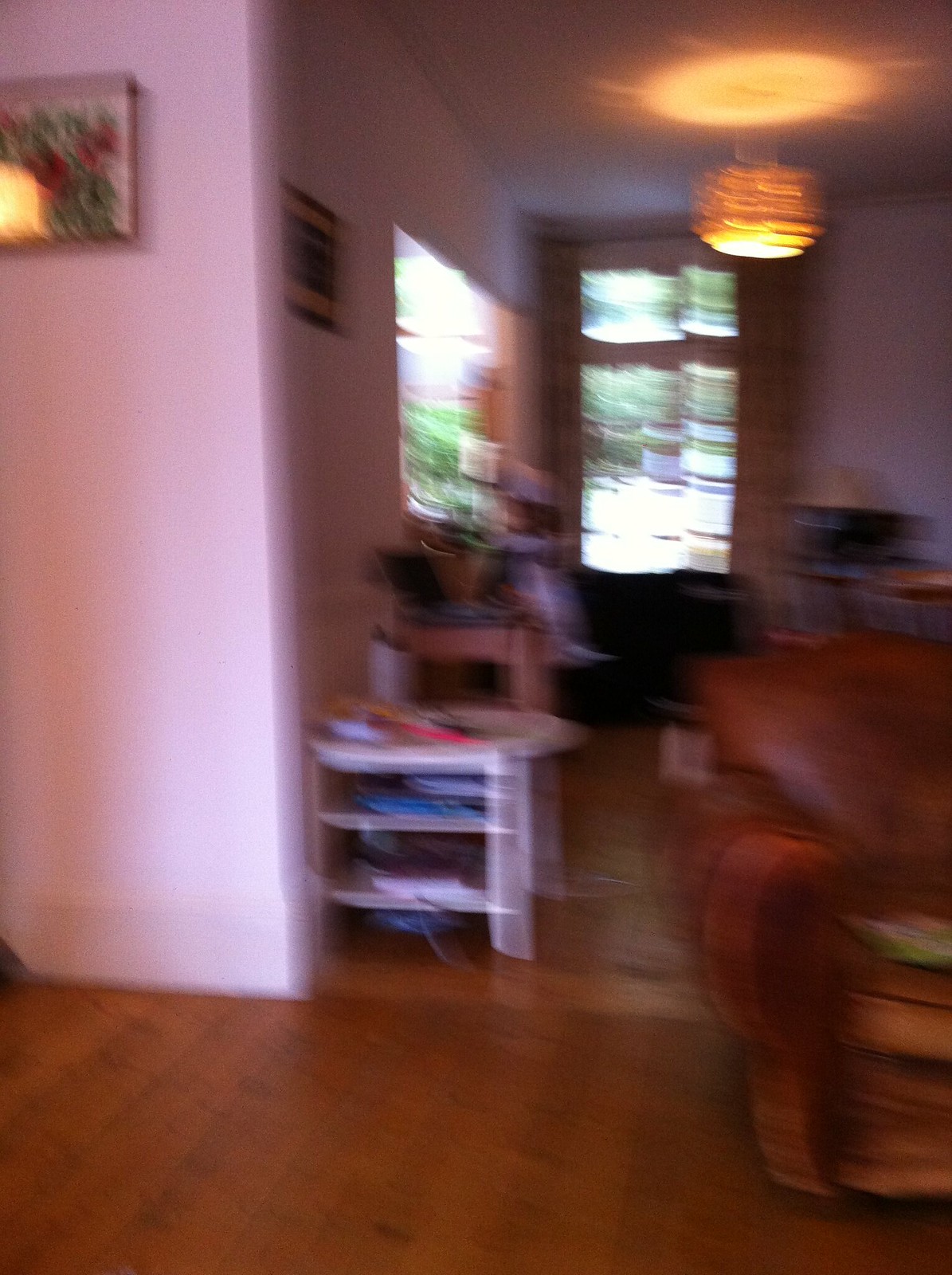The image is a blurry, diagonal, indoor color photograph of a living room taken with motion, resulting in a low-quality, dark, and disproportionate view. The room features a dark brown hardwood floor and white walls, one of which has a picture reflecting an orange-tinged ceiling lamp, casting an orange circle. Near the center, partially obstructed by a brown leather couch, stands a cluttered white side table with multiple levels for storage. Additional furnishings include a comfortable-looking large orange-brown leather chair with clothing draped over it and another brown table next to the white one. In the distant corner, a computer is visible, and tall windows frame the background. A prominent circular light chandelier hangs from the ceiling, contributing to the room’s illumination. The overall scene appears cluttered and somewhat chaotic due to the photograph’s poor quality and motion blur.